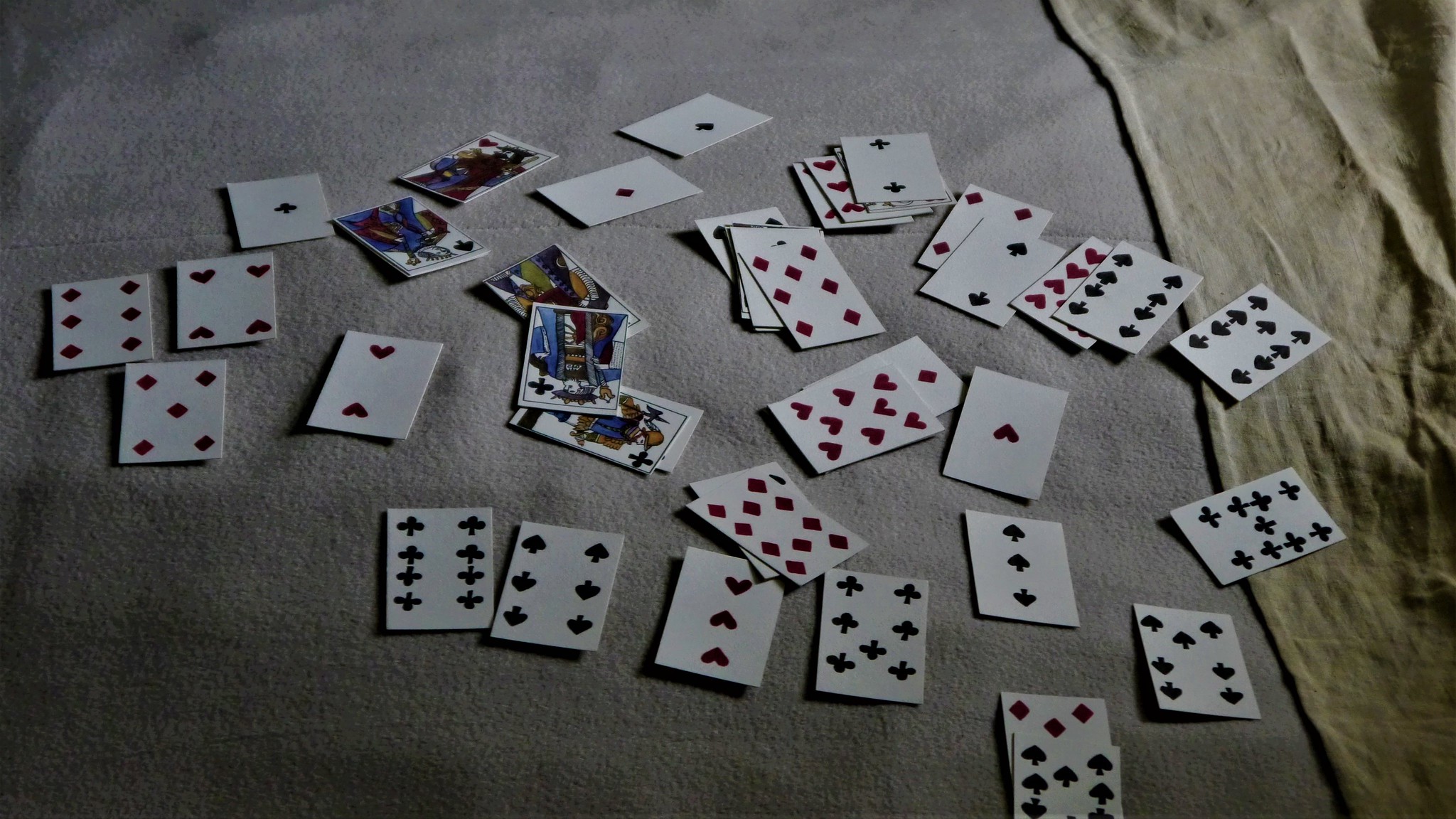This vibrant color photograph displays a seemingly haphazard scattering of playing cards across a surface, likely a table covered with a gray tablecloth. The tablecloth appears to shift to a light beige color on the right side, adding a subtle contrast to the scene. Among the cards, five face cards stand out prominently. The Jack of Clubs and the King of Spades are easily recognizable, while the other three face cards, though brightly colored, remain indeterminate. The scattered cards primarily belong to the clubs, hearts, and diamonds suits. Intriguingly, while the suits are visible, the numbers on the cards are not, adding a curious twist to the otherwise typical arrangement.